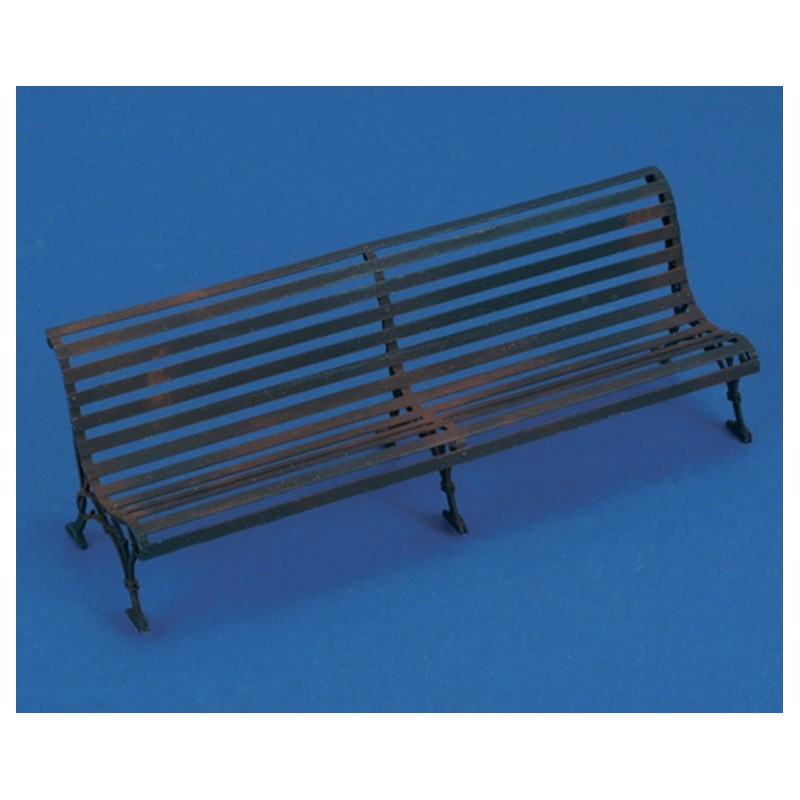This photograph features a weathered metal bench centrally placed against a uniform medium blue background. The bench, likely made of raw iron, is structured with metal pieces running across both the seat and slightly curved back, and it lacks armrests. The bench, which can accommodate approximately four to five people, has three sets of legs for a total of six legs. Each set, comprising two legs, is located at the ends and middle of the bench. These legs are slightly ornate and curved outward, adding a touch of design to the otherwise functional piece. The paint on the bench, originally black, has faded significantly, revealing patches of rust, particularly in the center and at the ends. This rusted and worn appearance indicates the bench has endured weathering over time.